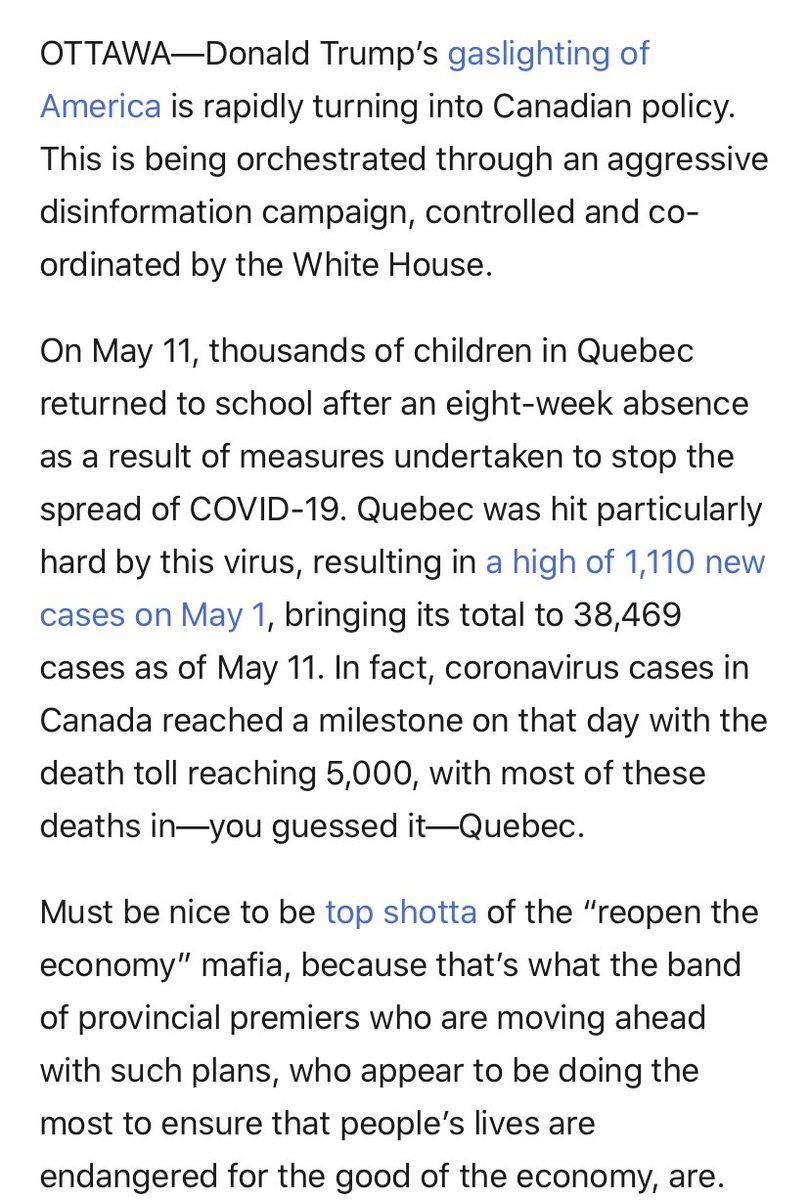Here is a cleaned-up and detailed caption for the described text:

---

The image features black text on a white background. The headline "OTTAWA" is presented in bold, capital letters. Below it, there is a highlighted line in blue that reads: "Donald Trump's gaslighting of America is rapidly turning into Canadian policy." This line is immediately followed by a detailed narrative explaining how an aggressive disinformation campaign, controlled and coordinated by the White House, is influencing Canadian policy.

After a paragraph break, the text continues by discussing the impact of COVID-19 in Quebec. It notes that on May 11, thousands of children in Quebec returned to school after an eight-week absence due to measures aimed at curbing the spread of the virus. Quebec was severely affected, reporting a peak of 1,110 new cases on May 1 (this figure is also in blue), bringing the province's total cases to 38,469 by May 11.

The narrative goes on to state that on the same day, Canada reached a significant milestone with the national COVID-19 death toll hitting 5,000, the majority of these deaths occurring in Quebec.

A new paragraph begins with the sentence, "Must be nice to be the top shotta of the 'reopen the economy' mafia." Here, "top shotta" and "reopen the economy" are emphasized in blue. This section critiques the provincial premiers pushing to reopen the economy, suggesting they appear to prioritize economic gains over public health.

At the end of each line in the image, specific words are noted before a space or paragraph break: "policy, aggressive, co, house," followed by a space, then "Quebec, absence, the, particularly, new," then the number "38,469." Further, it lists: "In the, these, Quebec," another paragraph space, and finally, "the, band, ahead, the, are, are."

---

This cleaned-up caption maintains the essence and details of the original narrative while ensuring clarity and readability.